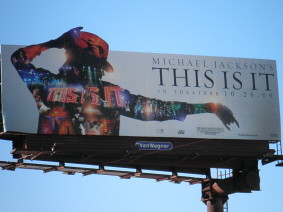The image features a billboard set against a sky blue background. The billboard is mounted on a brownish post or frame, which includes a blue label with white writing. The main billboard is white and displays a striking silhouette of Michael Jackson, adorned with a hat. One of Michael's hands rests on the back of his hat, while the other is extended forward in a dynamic hand gesture. Within his silhouette, vibrant lights, performers, and dancers add a colorful and lively scene. At the top right corner of the billboard, the text reads, "Michael Jackson's This Is It in Theaters," followed by a partially visible date that appears to be "10/24/09."